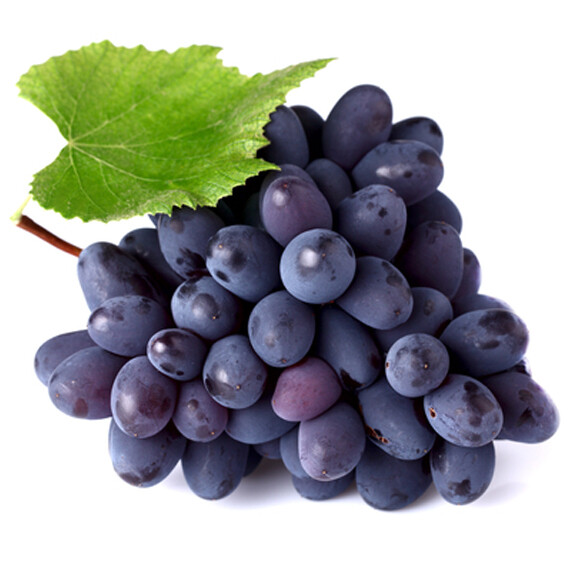This is a detailed photograph of an abundant bunch of dark purple grapes, reminiscent of Concord grapes, tightly packed in a pyramid shape. Approximately 40 to 50 grapes are connected by a central vine, which culminates in a small, visible stem on the left side. Atop the mass of grapes rests a single green leaf, adding a touch of contrast to the cluster. A few of the grapes feature darker spots, potentially indicating slight decay, and some exhibit a yellowish shine from the lighting. The background is a stark, clean white, placing full emphasis on the rich, deep-blue hues of the grapes, highlighted by some redder, not-quite-ripe variations.